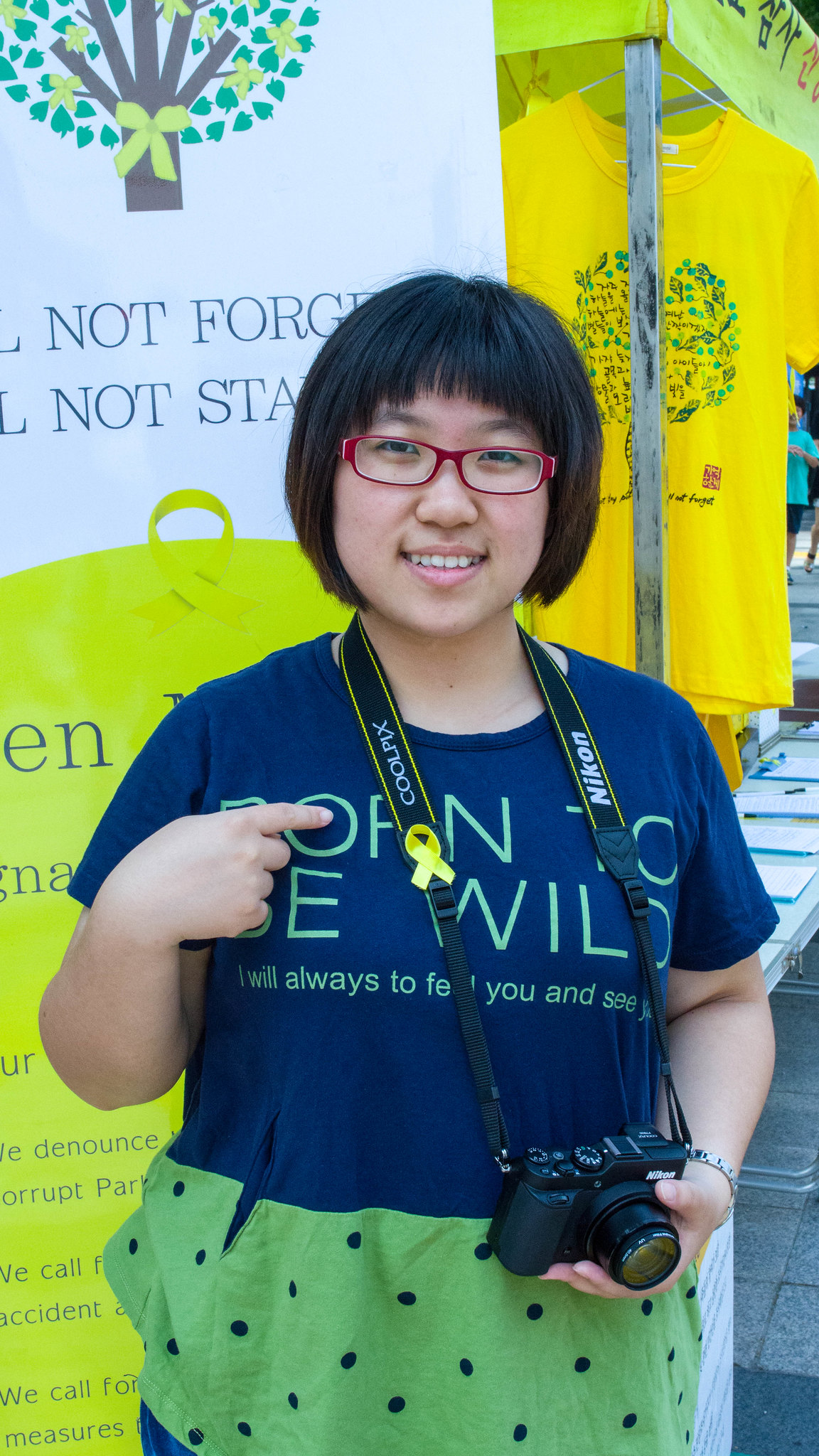In this vibrant and dynamic image, a young woman, approximately 18 or 19 years old, is the focal point. She has short bobbed, black hair and wears stylish red-framed glasses. With a cheerful smile, she looks directly at the camera, which she holds in her left hand, the Nikon camera suspended around her neck on a strap with noticeable yellow lines and a yellow ribbon. The woman's attire features a unique, blue short-sleeved shirt adorned with light green text that reads, "Born to be wild, I will always feel you and see you." Her right hand playfully places her pointing finger inside the "O" of the word "Born." The lower portion of her shirt transitions to a light green shade with blue dots. 

Behind her, various elements lend a vivid background to the scene. To the left, partially obscured by the woman, stands a sign with a graphic of a tree and a ribbon, featuring the words "Will not forget," although some text is not fully visible. Hanging on a pole to the right is a yellow t-shirt. Further off in the background, to the right of the yellow shirt, a man can be seen wearing shorts and a light blue shirt. The ground appears to be made of stone brick, suggesting an outdoor setting, possibly at a street vendor area or an outdoor festival, where the main colors—yellow, blue, green, and white—blend seamlessly, creating a lively and colorful atmosphere.